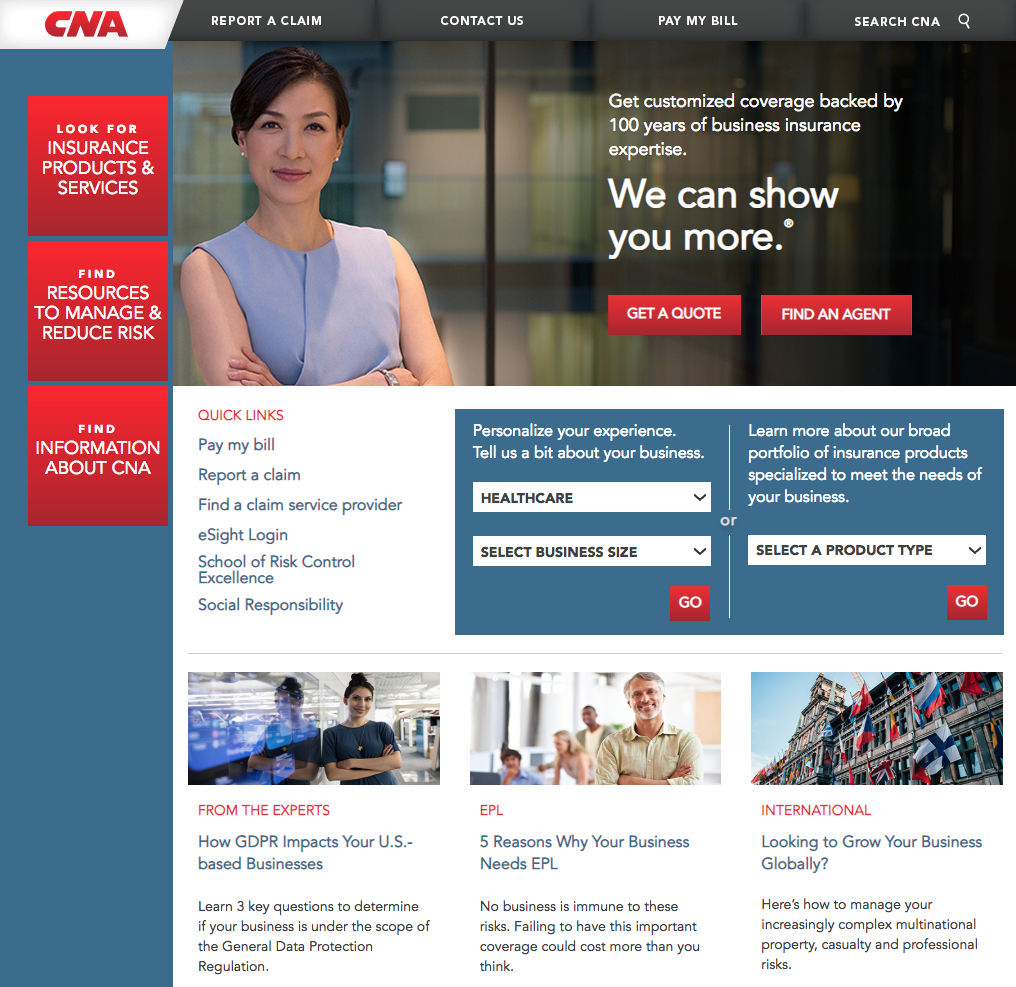This image appears to be a screenshot from a website, likely the homepage of an insurance company. The upper section of the webpage features a rectangular banner with navigation options, including "Report a Claim," "Contact Us," "Pay My Bill," and a search bar labeled "Search CNA." At the top, the company's name is prominently displayed in red, although part of it is obscured in the image.

On the left side of the screenshot, there are three distinct vertical boxes. The first box prompts visitors to "Look for Insurance Products and Services." The second box offers resources to "Find Resources to Manage and Reduce Risk." The third and final box provides information under the heading "Find Information About CNA."

Central to the image is a photograph of a woman dressed in a purplish sleeveless dress, with her hair neatly pulled back. She is smiling softly without showing her teeth. Adjacent to her image, a text overlay reads, "Get customized coverage backed by 100 years of business insurance experience." Below this, the text suggests, "We can show you more." There are also interactive options presented, including a button labeled "Get a Quote" and a link to "Find an Agent."

This detailed screenshot reflects the website's user-friendly interface, designed to guide visitors through various insurance-related options and services with ease.